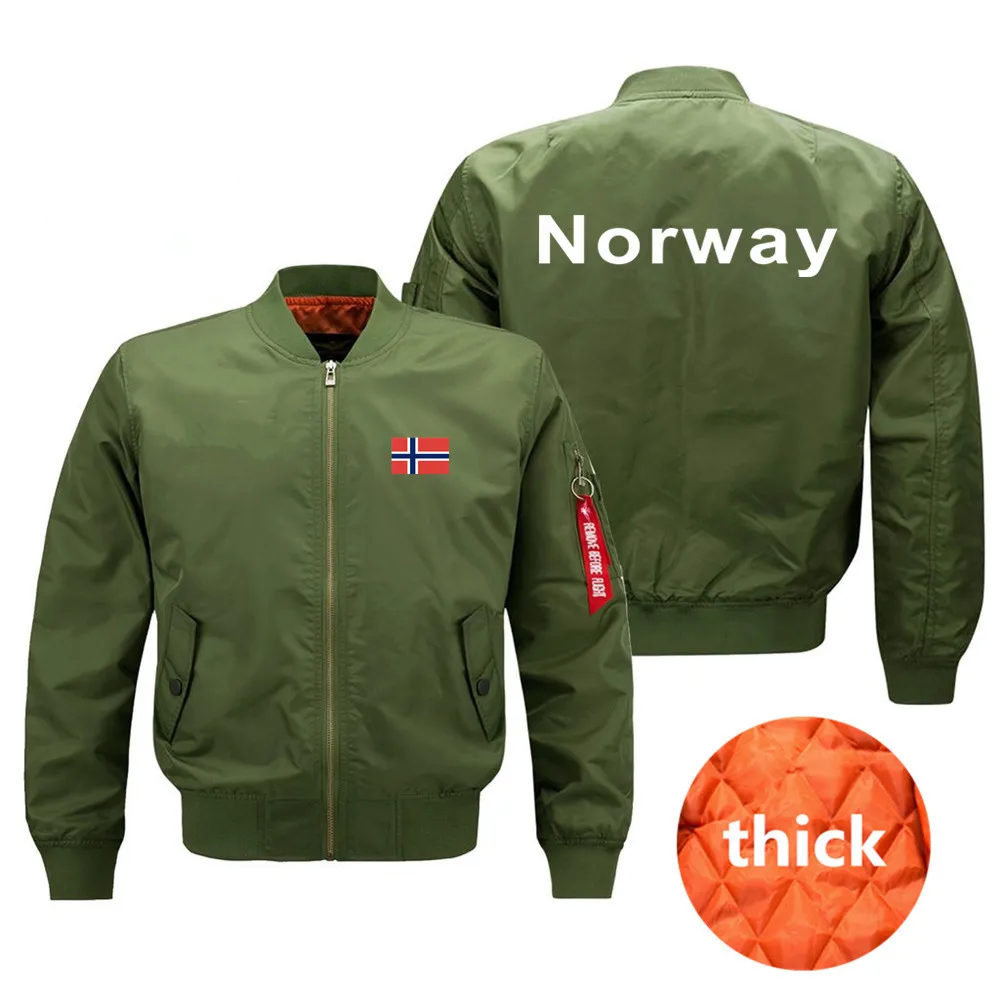The image depicts a green jacket with both its front and back views against a white background. The front view, positioned slightly to the center-left, showcases a green jacket with a red interior, a central zipper, and two pockets. On the right chest area, there's a rectangular Norwegian flag featuring a red background with a dark blue cross bordered by white. On the left sleeve near the shoulder, a red keychain or tag with white text is attached. The back view of the jacket prominently displays the word “Norway” in white letters. Additionally, a circular inset located at the lower right of the image zooms in on the inner lining’s orange, rhombus-like quilted pattern with the word “thick” written in white sans-serif font. This setup presents the jacket as a fashionable apparel item, almost resembling a bomber jacket, with a distinctive military green shade.